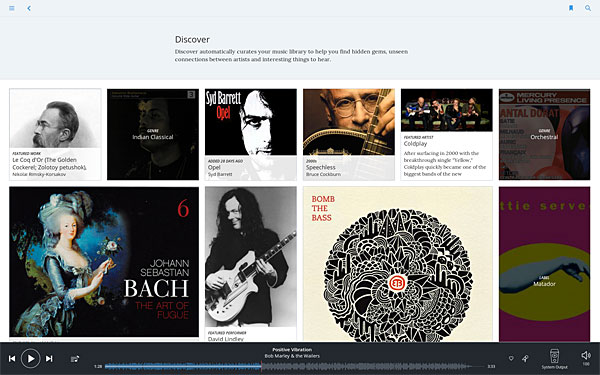The image can be described in the following detailed caption:

At the top of the image, a long, light blue rectangle spans horizontally with the word "Discover" prominently displayed in black text. Below this section, on the left, there is a black and white photograph of a man's profile. The man, who has glasses and a mustache, appears in a side view. Moving to the right, the next section features an image of Sid Barrett, also in black and white. Adjacent to him is another black and white image, this time of a man wearing glasses and holding a guitar.

Further to the right, there is a reference to the band Coldplay. The bottom row starts with a picture of Marie Antoinette on the left, with the number six displayed in the upper corner. Next to her image stands Johann Sebastian Bach, followed by an image of a man holding an electric guitar, smiling, with long, dark hair, in black and white.

The next segment in the upper left corner features the phrase "Bomb the Bass" in red text. Following this, there is an image inside a circular frame, displaying various flower petals in black and white. To the right of this circular image, there is a combination of a pink background with a yellow circle inside. Additionally, there is a visual of a blue arm.

At the very bottom of the image is a long gray rectangle, equipped with controls offering the option to play, fast forward, or rewind the content.